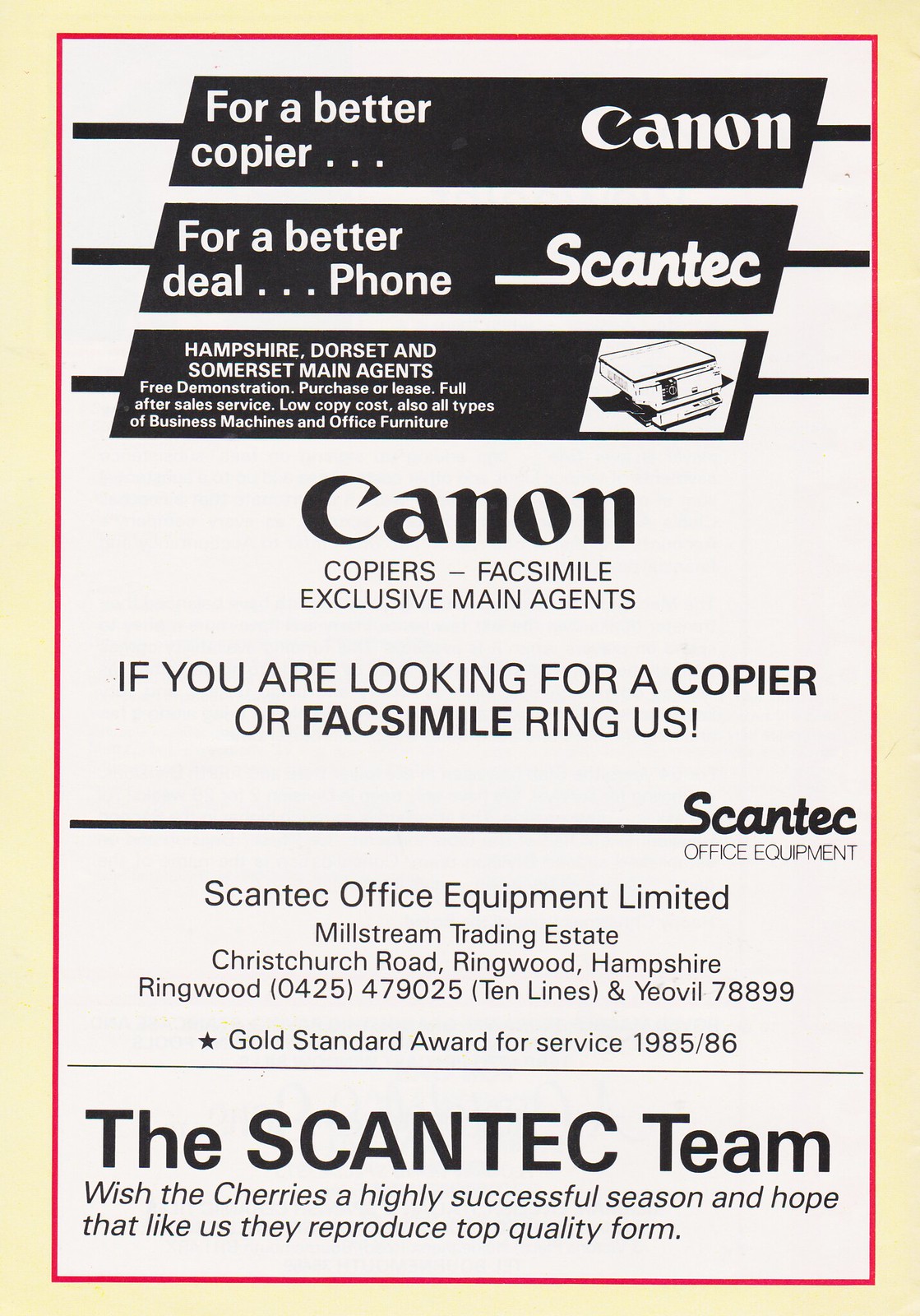This vintage advertisement features a black and white design with a red border, displayed on a white background. At the top, three black banners with white text stretch nearly across the width of the piece. The first banner reads "For a better copier, Canon," while the second states "For a better deal, phone Scantech." The third banner includes smaller, more detailed text mentioning "Hampshire, Dorset, and Somerset main agents," "free demonstration," "purchase or lease," "full after-sale service," "low copy costs," and "all types of business machines and office furniture," next to an illustration of a Canon copier.

Prominently below these banners, bold text declares "Canon copiers, facsimile, exclusive main agents." It continues, "If you're looking for a copier or facsimile, ring us." Further down, it lists "Scantech Office Equipment Limited," along with their address and phone number. At the bottom, a supportive message says, "The Scantech team wishes the Cherries a highly successful season and hopes that, like us, they reproduce top quality form."